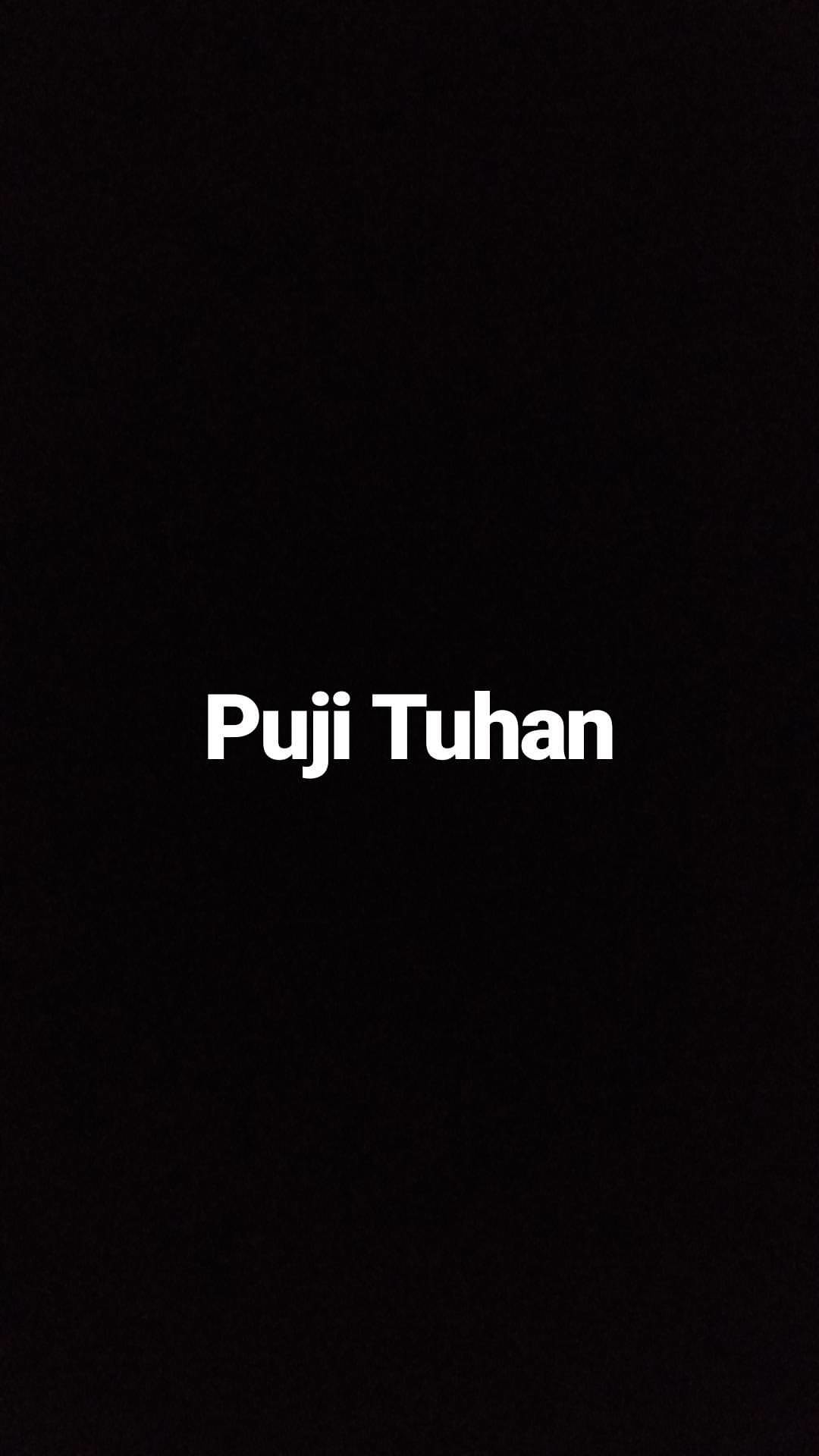The image is a simple yet striking design featuring a vertically-oriented, solid black background. In the exact center of this portrait-oriented rectangular frame, two words are boldly displayed in a white, sans-serif font: "PUJI TUHAN." The text is written in capital letters, with "PUJI" on the top and "TUHAN" directly below it, creating a clear and focused visual statement. There are no additional symbols, images, or textures, making the contrast between the black background and the white text the focal point of the image. This minimalist approach emphasizes the text, which appears to be in a different language, adding a layer of intrigue and clarity to the otherwise stark and simple composition.